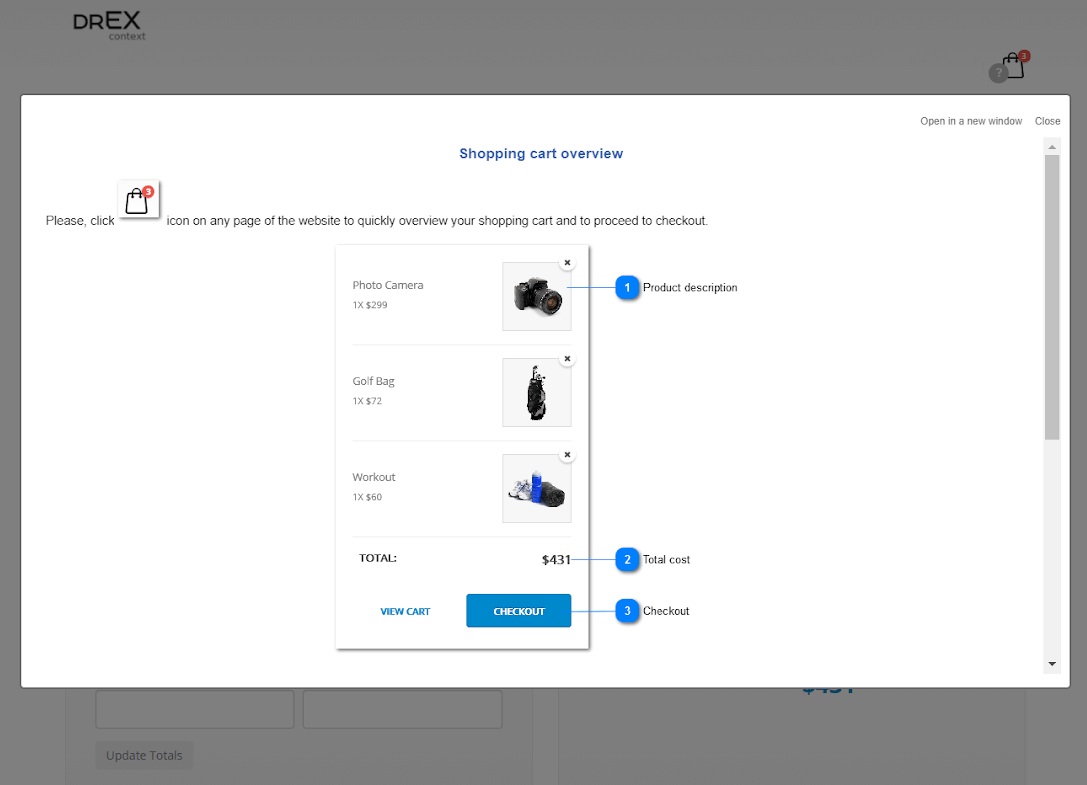The screenshot from a website, presumably named "Drex" (with the 'E-X' portion of the name prominently larger than 'Dr'), features a grayed-out background that is partially transparent, allowing glimpses of the underlying webpage. Central to the image is a prominent white pop-up window with a title reading "Shopping Cart Overview," despite the presence of a shopping bag icon in the top-right corner of the site. This icon, accompanied by a question mark or info button, displays a red circle indicating the number of items in the shopping bag.

The pop-up window details the contents of the shopping bag, listing three items, each with a thumbnail image, product name, price, and brief description. The first item is a photo camera, with its description and thumbnail to the right. The second item is a golf bag. The third entry shows workout shoes and a water bottle, suggesting a set or combo deal. The cumulative total cost of these items is displayed as $431.

Below the itemized list, the interface offers a "View Cart" option and a prominent blue "Checkout" button, reinforcing the usability and accessibility for completing purchases. This screenshot appears to serve as an educational or demonstrative example illustrating how an e-commerce shopping cart can be visually and functionally structured within a website using the Drex platform.